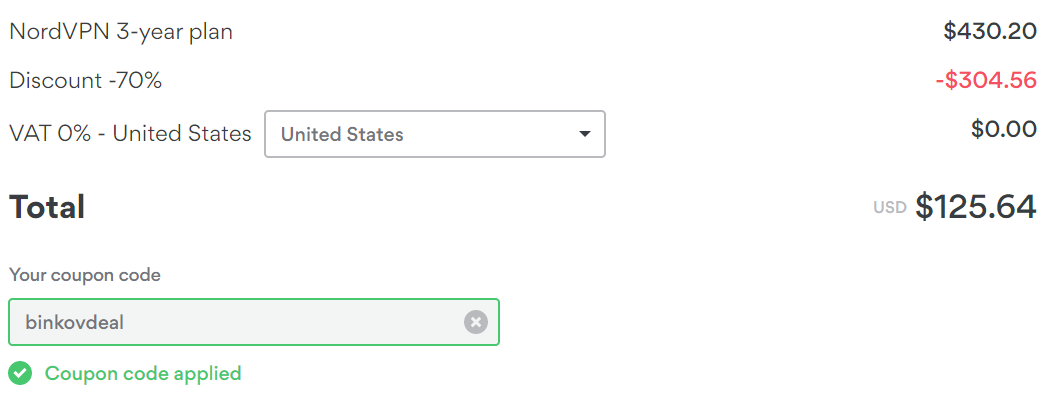This horizontal image displays a complex billing summary with various text fields, values, and colors. On the left side in gray font, "NORDVPN3-Year Plan" is written, detailing the subscription plan. On the extreme right side in black font, the cost of the plan is specified as "$430.20". Further to the left, there is a "Discount - 70%" section in gray font. Adjacent to this, in red font, is the discount amount, represented as "-$304.56".

Returning to the left, there is a section in all capitals: "VAT0% - United States." Below this, there is a dropdown field with "United States" pre-selected. To its right, "$0.00" is displayed, indicating no additional VAT charges.

The "Total" amount is emphasized in bold black font with "USD" indicated in small capital letters beside it in gray font. The final total cost is presented in bold black as "$125.64".

Moving back to the left side, a small-font label reads "Your Coupon Code". Below this label, there is a bright green-outlined field containing the coupon code "BinkoVDeal" as a single word. On the right side of this field is a white "X" in a gray circle, indicating the option to remove the coupon. Underneath, a green circle with a white check mark and the text "Coupon Code Applied" confirm the successful application of the discount.